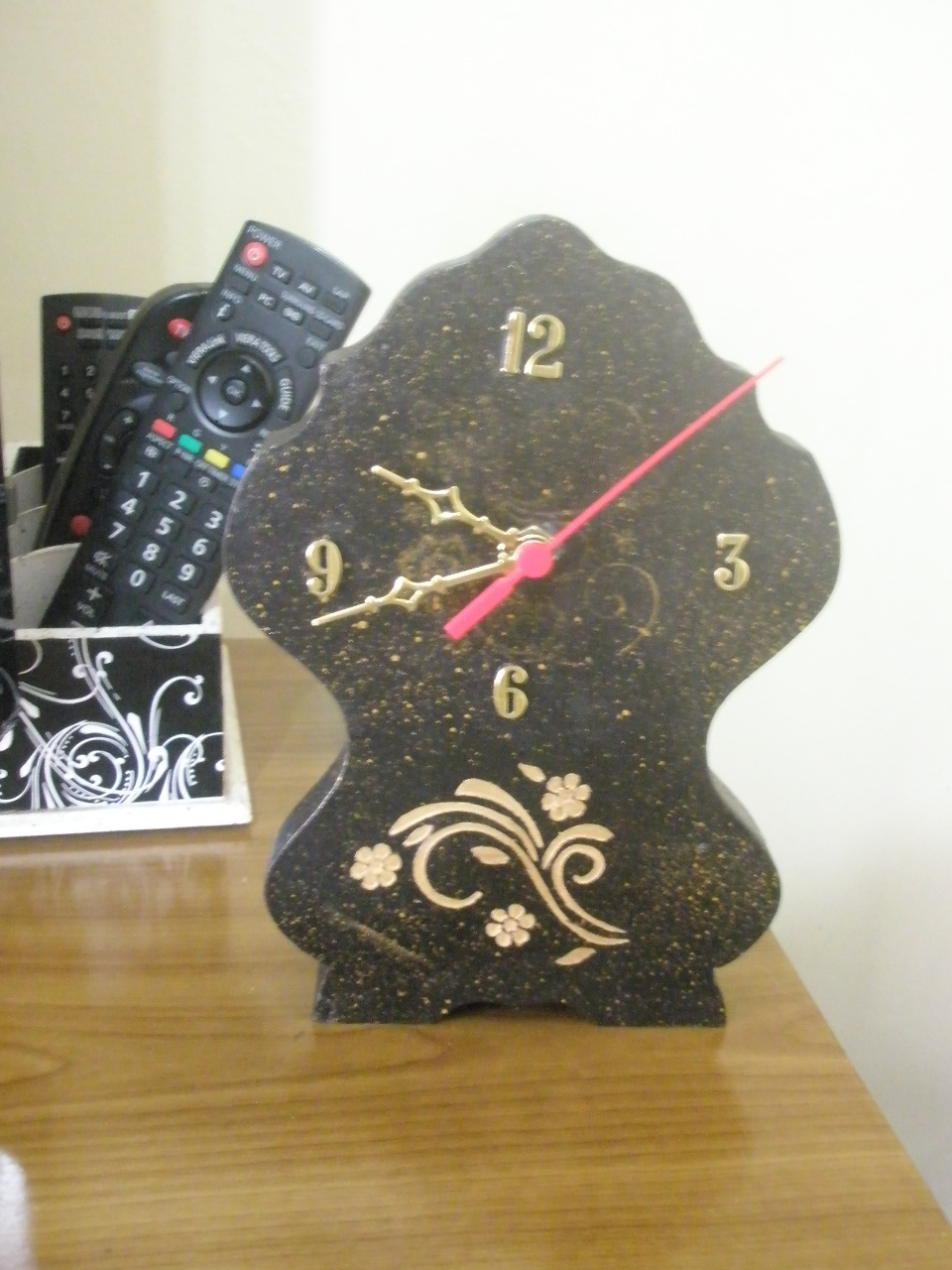In this vertically oriented rectangular photograph, a clock is prominently displayed on a wooden brown table. The clock face shows the time as approximately 9:44. It features two elegant gold hands, adorned with a small diamond at their intersection, and a distinct pink second hand that is pointing towards the 10 o'clock position. Only the numbers 12, 3, 6, and 9 are marked on the clock face, all in gold. At the bottom of the clock face, there is a decorative flower-like symbol. The entire backdrop of the clock face is solid black, accented with scattered gold specks. Adjacent to the clock, also on the table, sits a white tray or cart, which holds a collection of black TV remotes.